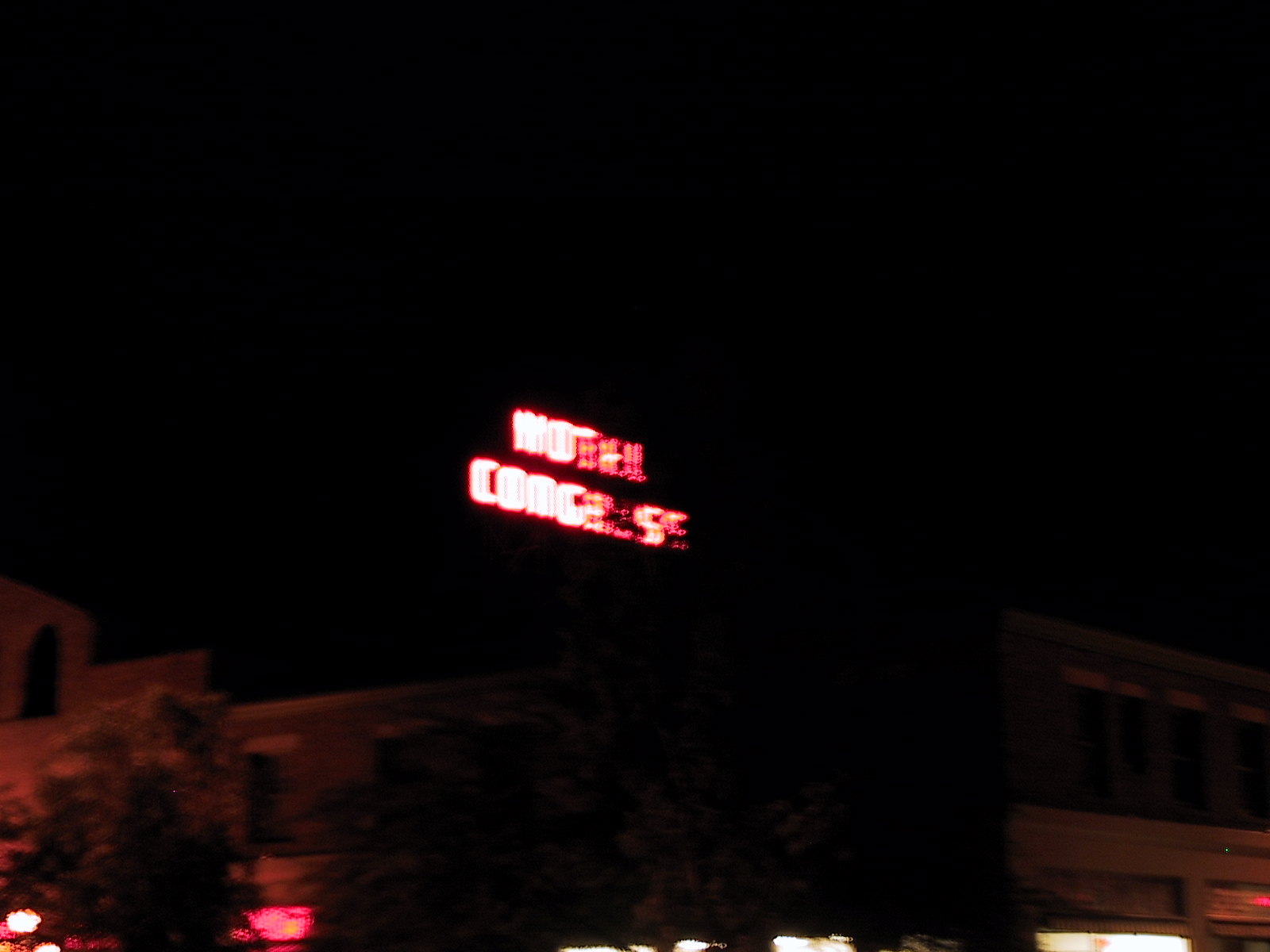This photograph, blurred and taken at night, captures an outdoor scene dominated by a black background, with the faint outline of a large masonry building barely visible in the lower left corner. The edifice, partially obscured by some trees, features a mix of white and red lighting at its base. Central to the image is a red neon sign that appears to be mounted on raised scaffolding above the building's roofline. The sign is illuminated with bright white light, though several of its bulbs have gone out, affecting the legibility of the letters. The top word likely reads "Motel," with the letters "M-O" brightly displayed while the rest are dim or unlit. Below, a second word starts with "C-O-M" or "C-O-A," followed by partially illuminated and unlit characters, suggesting it might spell out "Corcelese” or a similar name. The overall scene is enveloped in darkness, with the scattered white and red lights providing the only sources of illumination.